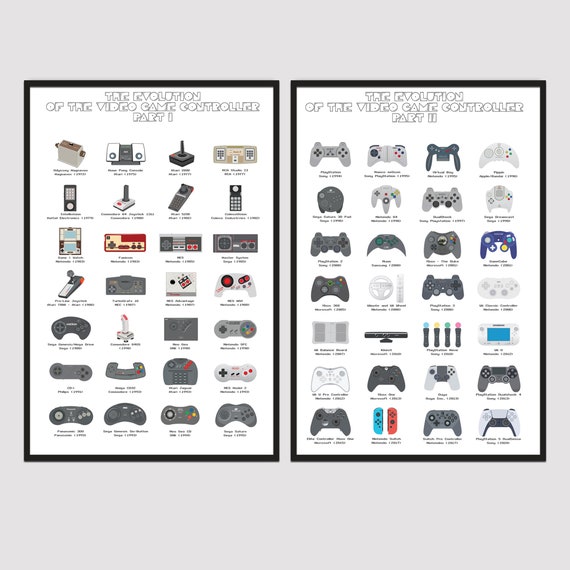The image features two side-by-side posters titled "The Evolution of the Video Game Controller Part 1" and "Part 2," each with a white background and a black frame. Both posters depict a comprehensive timeline of video game controllers, spanning from early models like the Atari and old Nintendo controllers to modern devices such as the Nintendo Switch, Wii, Xbox Series X, and PlayStation 5. Each poster arranges the controllers in a 7-by-4 grid, making a total of 28 controllers per poster. The controllers are illustrated with a primarily gray color scheme, punctuated by vibrant reds and blues depending on the model. Each controller is labeled, though the text is too small to be legible from a distance. Together, the posters provide a detailed visual history of video game controller evolution for both computers and gaming consoles.